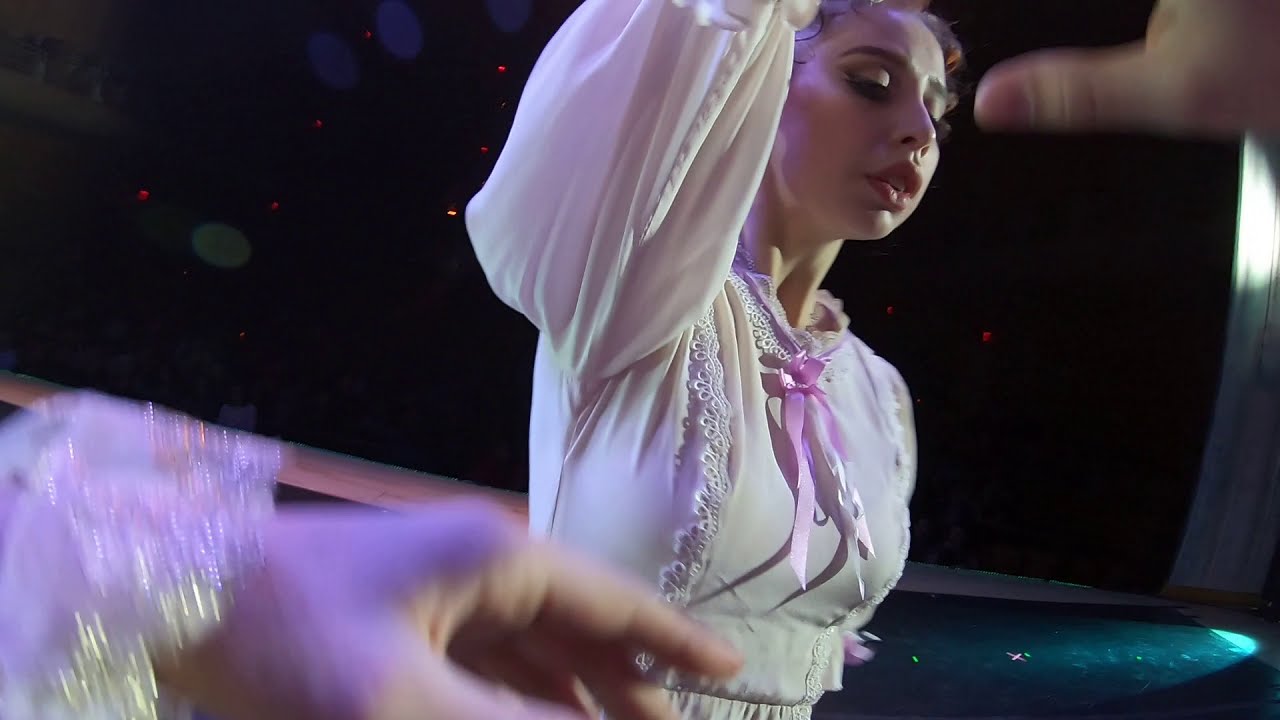The image depicts a scene that appears to be from a theatrical production, captured indoors. In the foreground, there is an up-close view of a female dancer, seen from the waist up. She is dressed in a white long-sleeve gown with intricate lace and gathers above the skirt, and she has a prominent purple (or pink) bow at her neck. Her hair is styled up, and she is adorned with heavy stage makeup that accentuates her full, round cheeks. Her right arm is raised, and she is seen in a right side profile with her eyes somewhat closed and her mouth slightly open, giving her a doll-like appearance. Framing her, we see parts of another dancer's arms—one with a frilly white sleeve and a cufflink in the lower left corner and a thumb in the upper right corner—suggesting the camera's perspective is from another dancer. The background is dark, possibly indicating a dimly lit stage, with a floor that appears to be dark green.